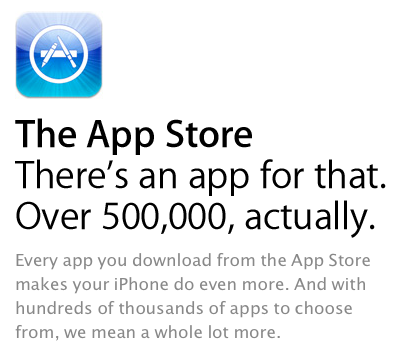This image appears to be a slightly wider-than-tall screenshot of a mobile-optimized website, likely focused on the Apple App Store. The background is white, presenting a clean and minimalistic design with primarily black text. In the upper left-hand corner, there is a square icon featuring a blue background with a white circle that encloses the letter "A," which strongly suggests it's the Apple App Store symbol. Confirming this, large bold black text beneath the icon reads "App Store." Below this heading, non-bolded black text proclaims, "There is an app for that, over 500,000 actually." Further down, in smaller, slightly grey text, it elaborates: "Every app you download from the App Store makes your iPhone do even more, and with hundreds of thousands of apps to choose from, we mean a whole lot more." The entirety of this text and imagery fits within a frame that is almost a square, slightly wider than it is tall, with no extraneous content visible. The upper edge is trimmed just above the top of the App Store logo, and the bottom edge is cut off just above the final line of text. The left margin is very narrow, less than a centimeter, while the right margin has slightly more space.